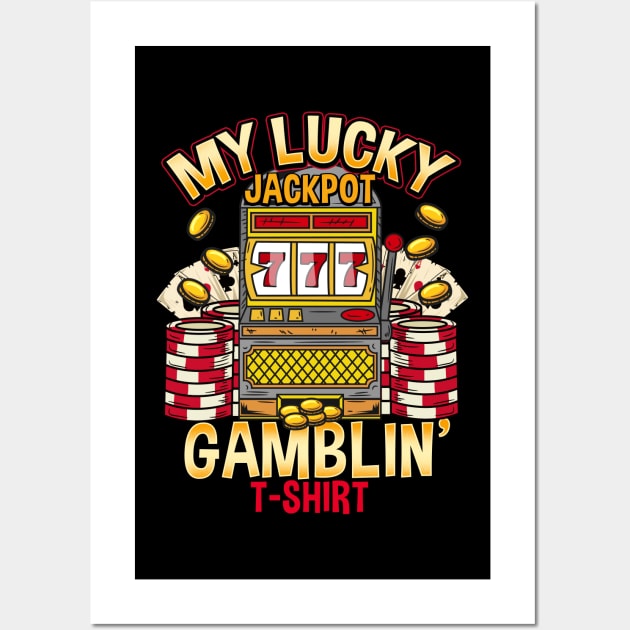This detailed illustration features a vibrant and colorful design centered around a slot machine emitting a classic casino vibe. The image is set against a black background with a prominent white border. At the top of the poster, in striking gold font outlined in red, the text reads "My Lucky Jackpot." Below the slot machine, the caption "Gambling T-Shirt," spelled out as G-A-M-B-L-I-N’ T-Shirt in red, delivers a playful touch.

The slot machine itself displays the winning combination of 777 in red, and it is accented by a red ball on the lever positioned on the right side. The machine includes three buttons, an oval bar, and a screen above the coin slot. Overflowing with gold coins, the slot machine presents a scene where coins seem to spill out and float in the air, adding to the sense of fortune. Alongside the slot machine, stacks of red and white poker chips, as well as playing cards—including aces—are meticulously illustrated, enhancing the gambling theme.

This colorful and detailed graphic captures the essence of casino excitement and luck, making it an eye-catching design for a t-shirt intended for avid gamblers.